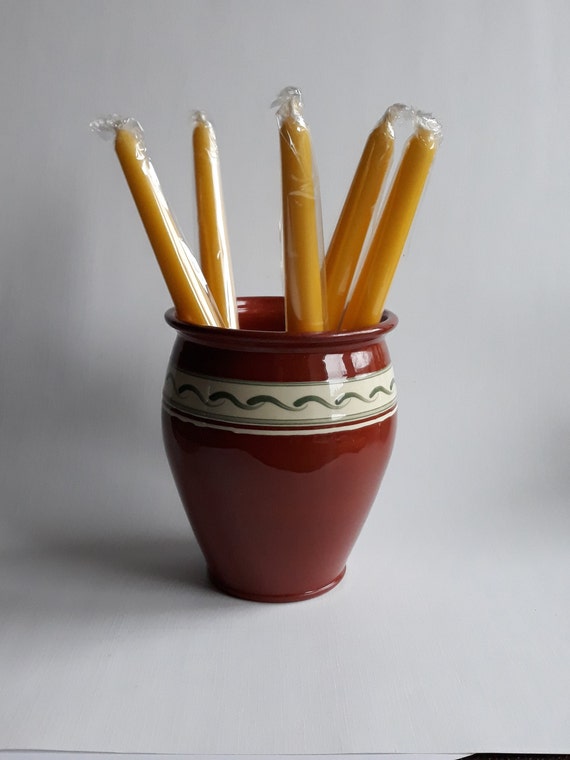This image features a glossy, dark-brown vase displayed on an off-white table. The vase, which has a highly reflective surface, tapers gracefully from a broad, round opening at its top to a narrower base. Adorning the upper three-quarters of the vase is a striking decorative ring, alternating between black and white in a snake-like, wavy pattern that adds a touch of intricate elegance to the piece. Emerging from the vase are five gold-yellow taper candles, neatly wrapped in clear cellophane plastic, with their wax and wicks visibly encased. The serene backdrop of an off-white wall complements the setting, highlighting the vase's unique design and the candles' rich hue.